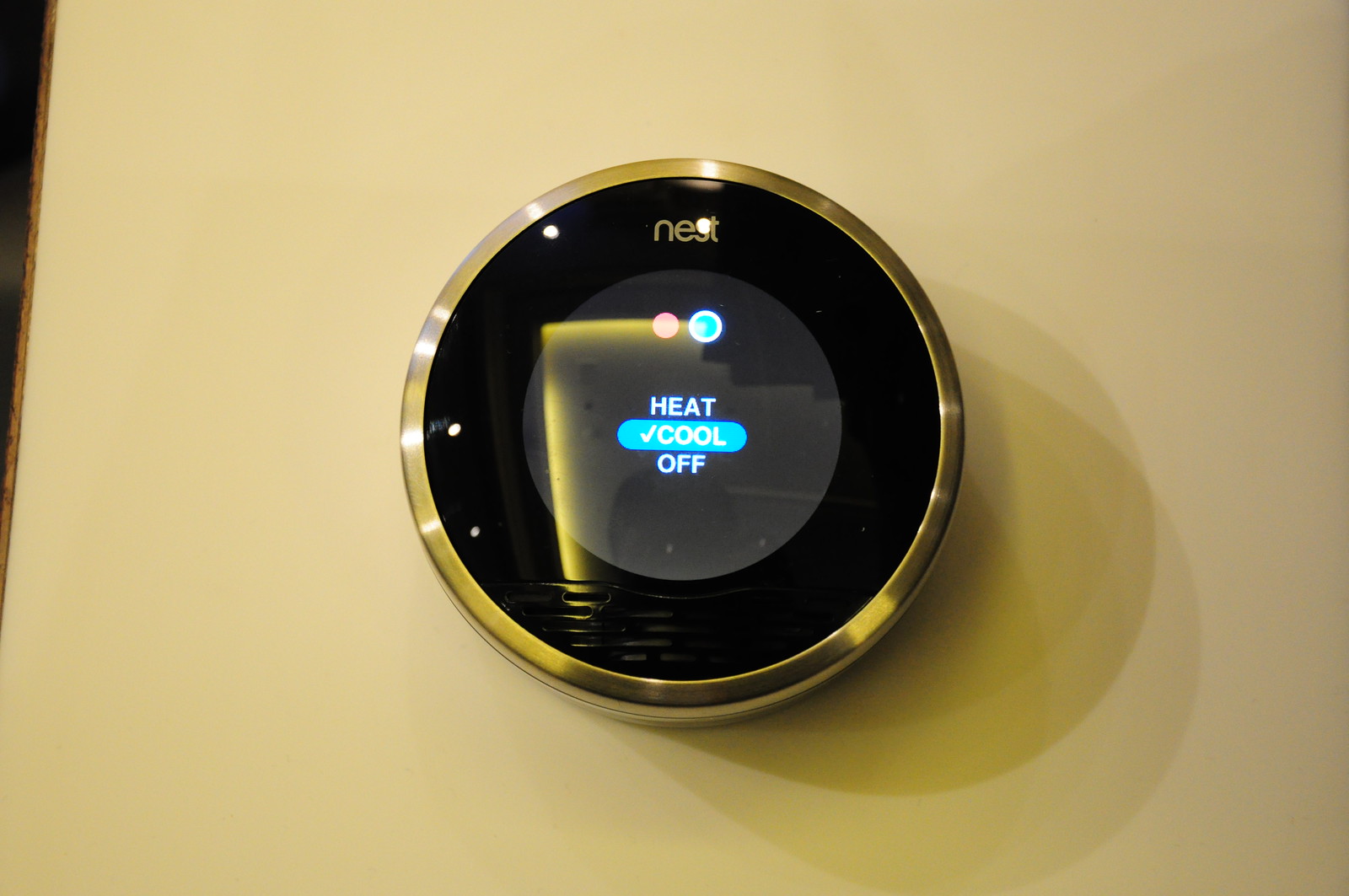The image depicts an elegant, high-tech thermostat mounted on a very light-colored, beige-pinkish wall. The thermostat features a brass-colored, circular frame with a glass front. Inside the glass, there is a thick black band with the brand name "NEST" prominently displayed in gold letters at the top.

Within the black band lies a gray circle, which contains further controls and indicators. Directly below the "NEST" branding, on the left side of the gray circle, there is a pink circle, while on the right side there's a blue circle rimmed in white. These likely signify different temperature settings or modes.

Toward the center of the gray circle, three words are displayed: "HEAT," "COOL," and "OFF." The word "COOL" is highlighted with a light blue capsule behind it, accompanied by a checkmark, indicating that the cooling mode is currently activated. This highlight matches the blue circle rimmed in white above it, possibly serving as an on/off indicator for the cooling function. The design and detail suggest a modern, user-friendly interface typical of a sophisticated smart thermostat.